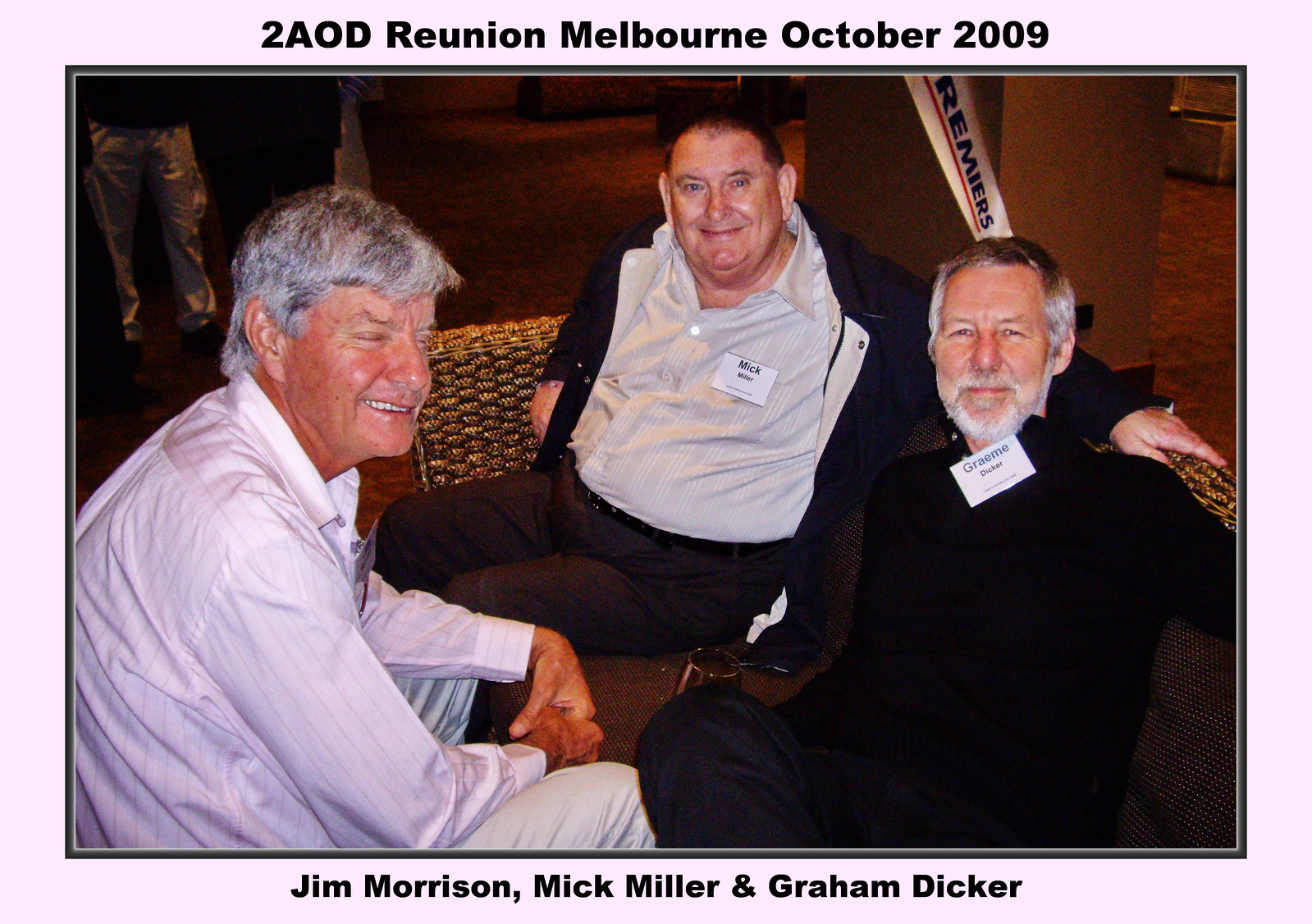The photograph captures a reunion event titled "2 A O D Reunion, Melbourne, October 2009," as indicated by the bold black text on a white background at the top of the image. The photo itself is horizontally arranged and enclosed by a pink border. At the bottom of the photograph, another caption in black text identifies the men as Jim Morrison, Mick Miller, and Graham Dicker.

In the foreground, three older Caucasian men are seated. The man on the left, identified as Jim Morrison, has thick gray hair and is clean-shaven. He wears a white button-down shirt open at the neck and tan trousers. Morrison is seated facing right, with elbows bent and forearms resting on his knees, hands crossed lightly in front.

The central figure, Mick Miller, is heavier and has a receding hairline with dark brown hair. He dons a black jacket over a white button-down shirt, tucked into dark gray trousers. Miller is smiling at the camera, with his left arm extended along the back of a sofa.

On the right, Graham Dicker has a full head of gray hair with a slightly receding hairline and a full gray beard and mustache. He is dressed in a black long-sleeve collared shirt, accompanied by black trousers. Dicker wears a white rectangular name tag at the upper neck area. Both Dicker and Miller's name tags are mentioned in the description.

In the background on the right side, a white rectangular column with a white banner reading "Remy" is visible. Additionally, the legs of three men standing and talking can be seen in the upper left corner, adding context to the social setting of the reunion event.